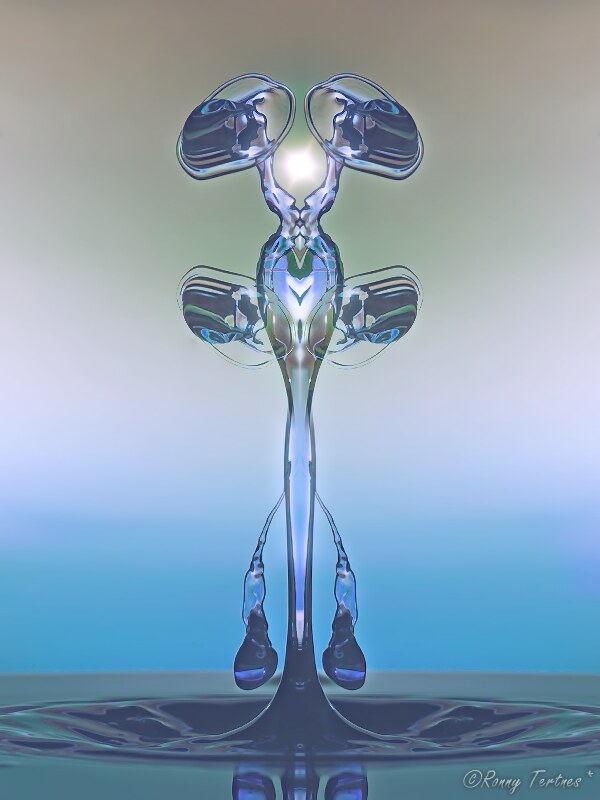In this image, we are presented with an artistic, digitally created poster that features a striking glass sculpture rising majestically from a body of water. This sculpture, primarily composed of clear and blue glass with purple hues, begins with a circular base that seamlessly transitions into a tapered glass form. From there, it expands into an oval shape and culminates with two arms extending outwards, each holding additional oval pieces of glass, creating a visually captivating design. The sculpture is centrally positioned within the image, accentuated by a background that transitions from a light blue at the bottom to a light white and finally to a light gray at the top, suggesting a gradient sky. At the base of the image, darker glass elements emanate from the main structure, adding depth and contrast. The scene is bathed in varying shades of blue, gray, and white, contributing to the ethereal and serene atmosphere. At the bottom right corner, a silver copyright mark reads "Ronnie Tertnes," indicating the author of this intricate artwork.